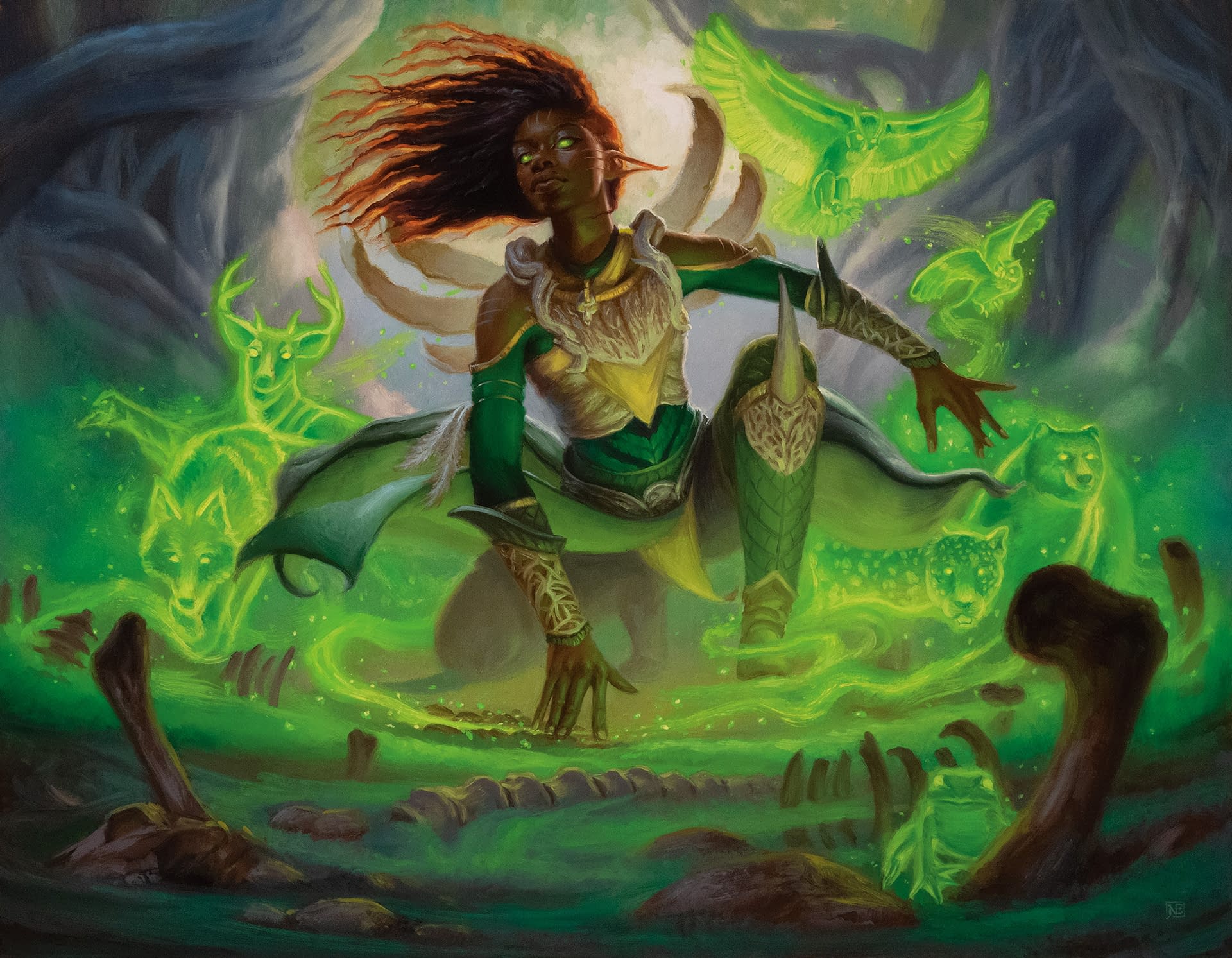The image is a detailed, computer-generated illustration of a formidable black female superhero who stands out vividly against a mystical forest backdrop. She has an athletic, muscular body with a very defined, sexy outline, and crouches in a powerful, pouncing stance, ready to engage her enemy. Her dark complexion is complemented by piercing green eyes and long, wavy, reddish hair that flows dramatically to the left. She has distinct pointy elf ears, and three rib-like white structures protrude from her back.

Her costume is predominantly green with gold accents, including medallions, breastplates, wrist guards, knee pads with outward-pointing horns, and a green cloak that flows behind her. The outfit is form-fitting like a tight shirt and leggings, but also has wing-like extensions resembling a skirt. Her right hand is planted firmly on the ground while her left hand is positioned behind her.

Surrounding her are ethereal, luminous green spirits of animals—a bear, a jaguar, a wolf, a deer, and an owl—each connected to her by swirling, glimmering lines of energy. These spectral creatures are positioned around her with the owl on her left shoulder, and the rest distributed on either side. A green, luminous squirrel and frog appear near the bottom right of the image, close to a misty foreground filled with animal bones. The backdrop features gray, curly tree trunks enveloped in a green mist, adding to the otherworldly and magical atmosphere of the scene.